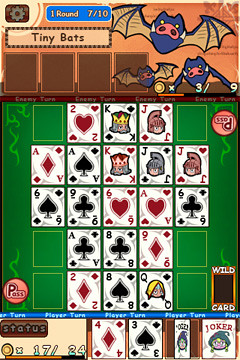This detailed caption provides a descriptive overview of a card game screenshot:

"In this card game screenshot, the interface showcases various game elements. At the top left corner, an icon for settings can be seen. The game is currently in round seven out of ten, indicated against a blue background adorned with tiny bats, with a few bats off to the side. The main game area includes four brown squares, each possibly representing different action zones or card placements. A coin counter shows '3/9' on the top right and '17/24' on the bottom left. There are wild card slots on each side, allowing players to make strategic plays from either side. A prominent pass button is available for the players. The player at the bottom holds a four of diamonds, a three of spades, and two jokers. The screen also displays numerous cards arranged in a 5x5 grid, suggesting a structured gameplay layout."